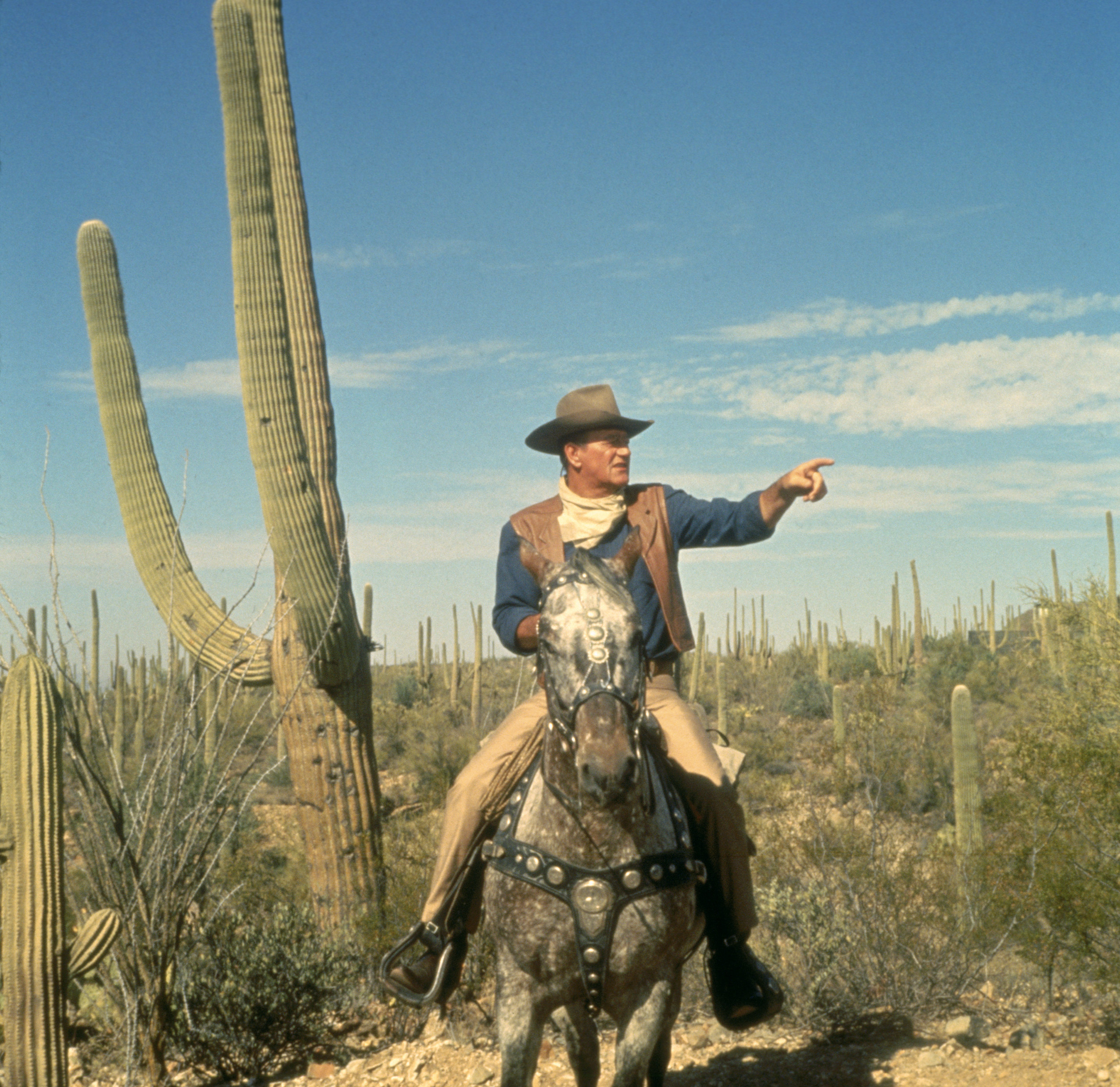The photograph depicts the iconic actor John Wayne, seemingly from a movie scene. Set in a sunlit desert landscape, the image shows Wayne mounted on a brown horse adorned with a fancy bridle and armor-like straps on its face and neck. Dressed in a cowboy hat, a blue collared shirt, a brown vest, and tan pants, Wayne is captured mid-action, pointing to the right of the frame with his left hand. The sun casts discernible shadows on the ground, and the backdrop features a clear blue sky with scattered clouds. To the left of Wayne is a towering cactus, approximately 15 feet tall, accompanied by several smaller cacti and desert vegetation, possibly San Pedro species, that enhance the arid ambiance. The scene exudes a classic Western vibe, likely from a movie poster or promotional still, emphasizing a sense of adventure and ruggedness characteristic of John Wayne's filmography.